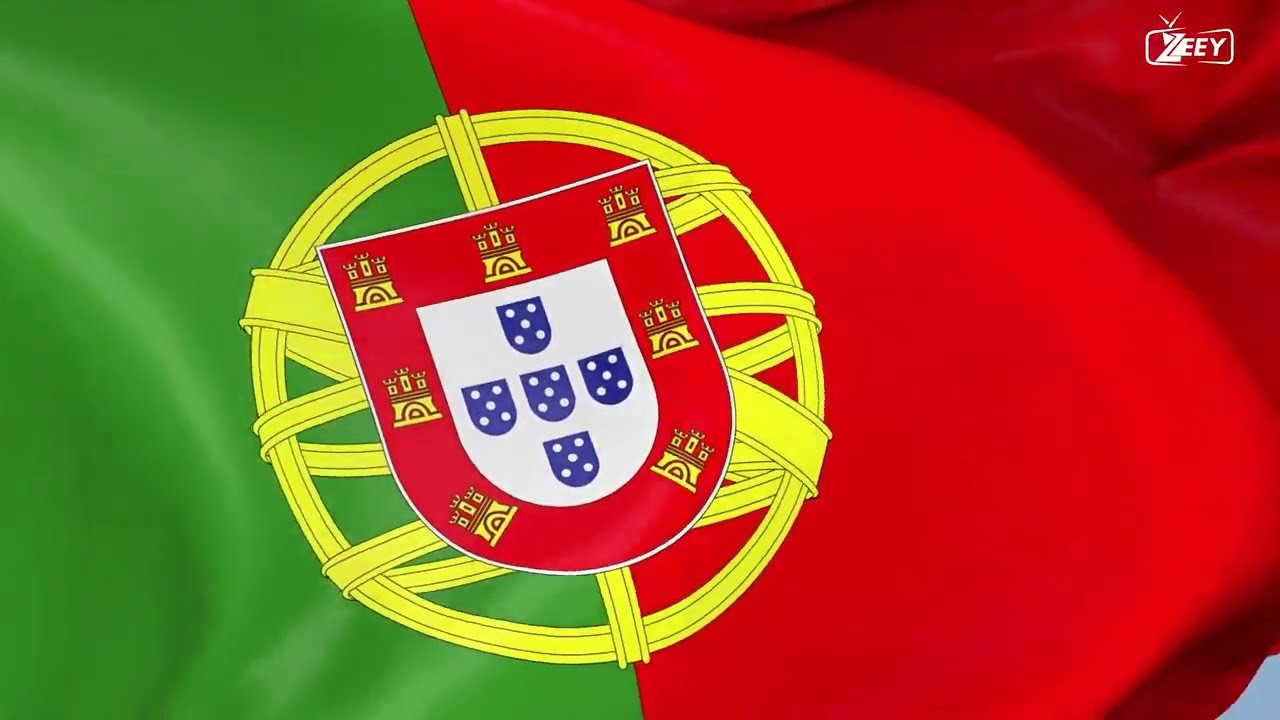The photograph captures a lively and intimate moment among five young Asian friends gathered around a circular table at an outdoor restaurant under a logo that reads "ZEEY." They're all fixated on a black smartphone being held by a man in a gray hoodie, who smiles as he shows something to the group. 

Seated next to him on the right is a woman in a bright yellow short-sleeved shirt with her long brown hair pulled into a ponytail, her arms folded on the table as she engages with the content on the phone. Leaning over her shoulder, a man in a gray shirt intently joins the viewing, bracing himself against a pole nearby. Behind the man with the phone, another person in a black and white striped t-shirt bends forward, curiosity evident on his face. On the left side, a man wearing a white button-down shirt with rolled sleeves beams while observing the screen.

The table they sit around holds coffee cups, suggesting they are enjoying a casual hangout, possibly after a meal, in wicker brown chairs. A vape and additional phones lie on the table, with the background showing other seating areas, reinforcing the relaxed, social atmosphere. Despite the various elements, the scene beautifully conveys a group of friends immersed in shared digital entertainment, embodying the essence of modern camaraderie.